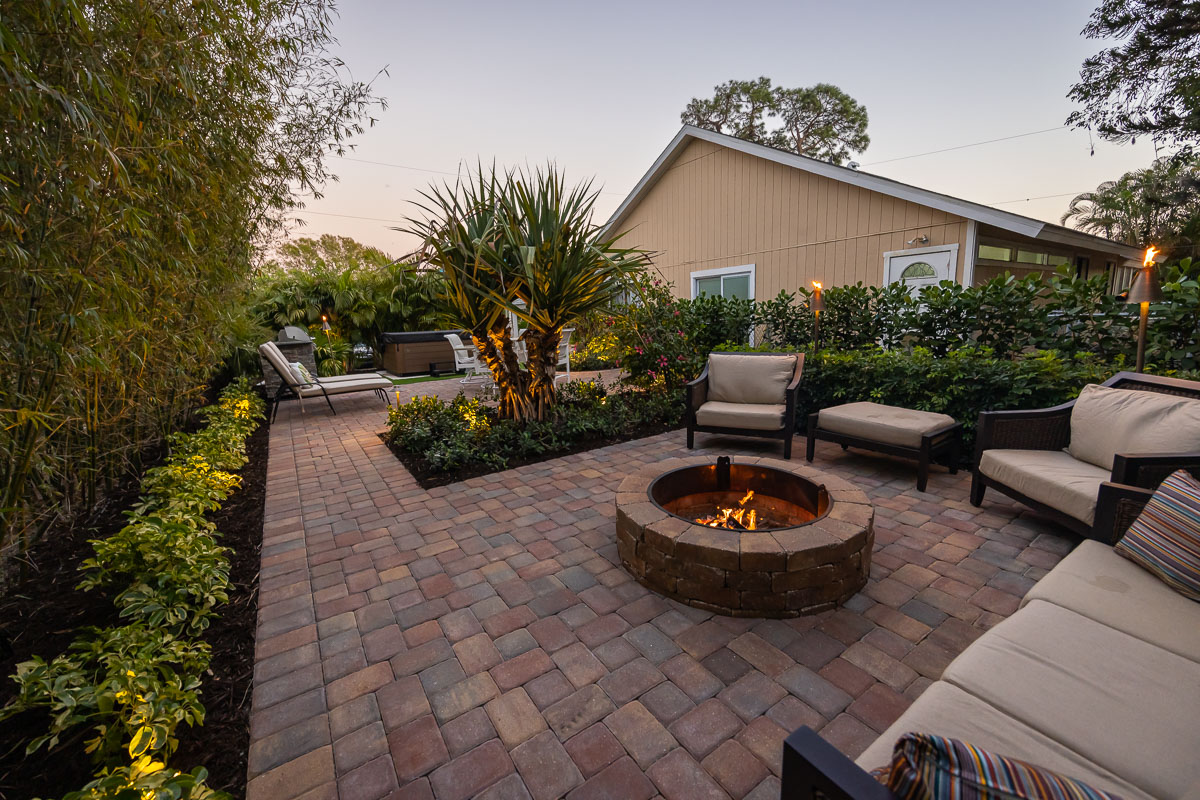This is a detailed photograph capturing the beautiful backyard patio of a single-story, ranch-style house bathed in the soft light of a sunset. The patio is composed of neatly arranged pavers in shades of brick red, tan, and gray. At its center is a small fire pit made of tan-colored bricks with a blazing orange fire. Surrounding the fire pit is an arrangement of cozy outdoor furniture, including black wrought iron chairs, ottomans, and sofas adorned with cream-colored cushions and striped pillows. The creamish light brown house, seemingly constructed of wood, forms the backdrop with its tan siding and white door.

On the left side of the patio, there's a mulch garden featuring green and yellow hostas and a screen of tall bamboo. Additional vegetation, well-maintained and strategically planted, borders the area along the fence. The garden is illuminated by decorative lights, adding a warm glow. Two brass-colored tiki torches also flicker in the foreground, enhancing the inviting ambiance.

A paved walkway, using the same pavers, connects to a separate patio area with matching wrought iron lounge chairs and a white dining table surrounded by white chairs. Palm trees and other lush vegetation suggest a warm, southern or tropical location, completing this picturesque and serene setting.